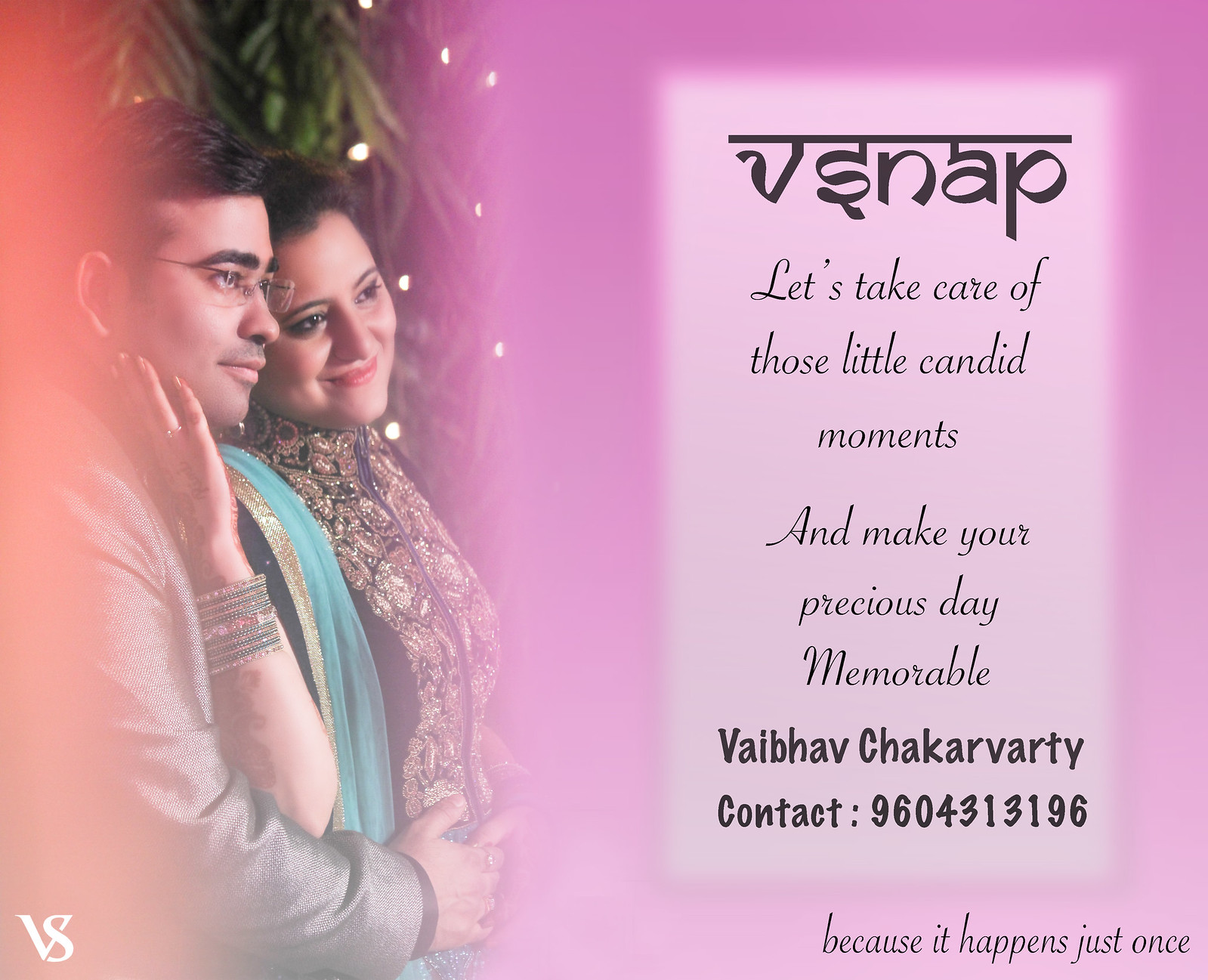In this color photograph, designed in a portrait orientation, a young Indian couple is featured on the left side of the image, smiling and embracing each other. The man, wearing a gray sparkly suit and wire-rimmed glasses, has his arms around the woman. The woman wears an elaborate, gold brocade Indian sari with a turquoise scarf draped across her shoulder, along with beaded armbands and a bracelet. They both look content, with the woman's hand resting on the man next to her, showcasing a candid moment of affection. Behind them, there's a backdrop of palm-like trees or ferns with a feathered edge, floating against a landscape-orientated purple background. 

To the right of the couple, the image transitions into a transparent white panel with black text. At the top is some text in an Indian language, followed by a scripted tagline that reads, "Let's take care of those little candid moments and make your precious day memorable." Beneath is the contact information for the photographer, Vaibhav Chakravarti, and a phone number, accompanied by the phrase, "because it happens just once." The lower left of the image also contains the initials "V-S." The overall style blends photographic realism with graphic design and typography, suggesting an advertisement for a photography company called V-Snap. The prominent colors in the image include purple, pink, black, tan, gray, light blue, and yellow.